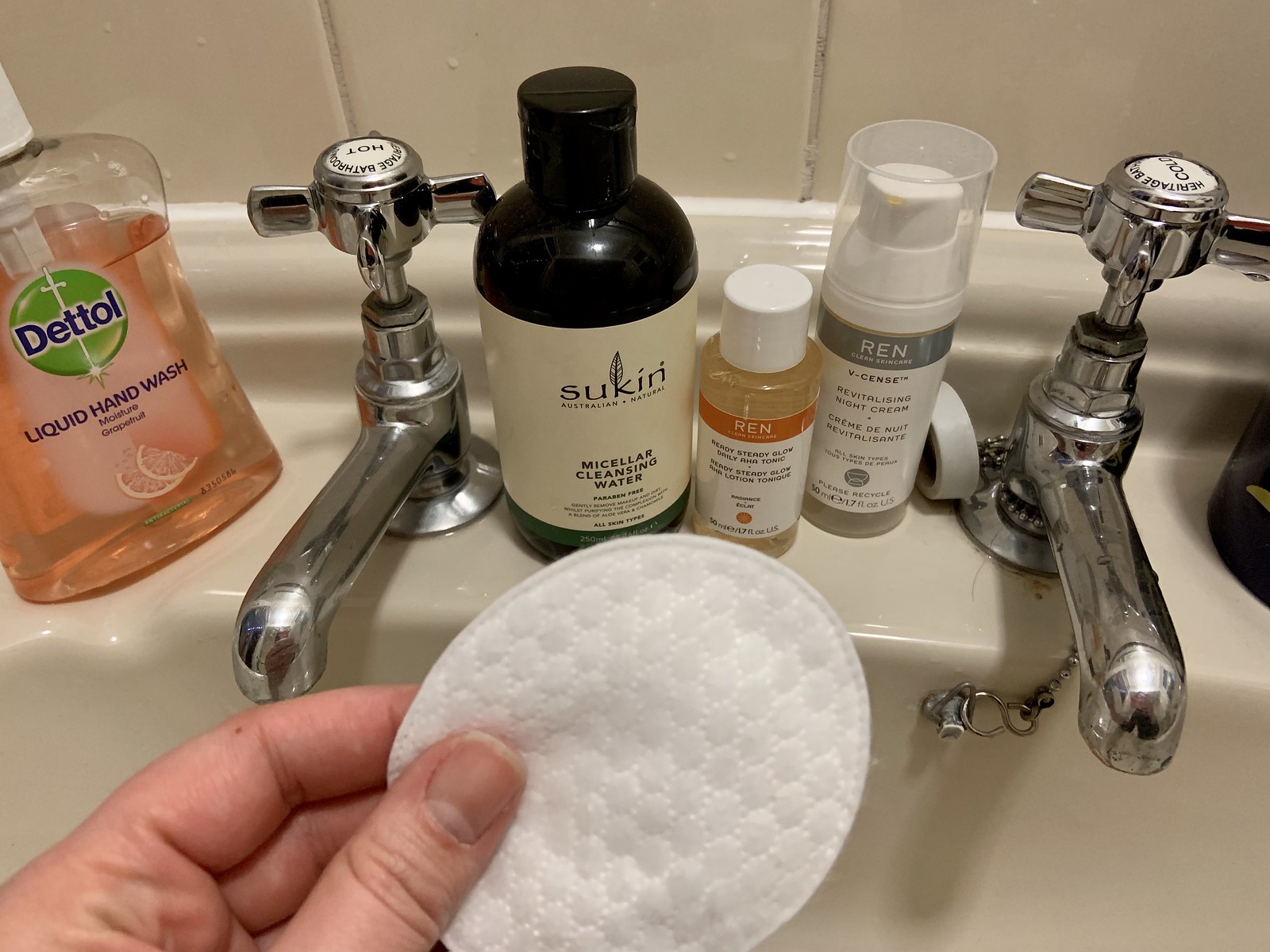In a cozy bathroom, a person is captured standing at a porcelain sink, holding an oval, padded makeup-remover pad in their left hand, with their thumb clearly visible. Centrally positioned on the creamy porcelain sink are three distinct bottles. Two of the bottles belong to the brand Wren, while the third, a sleek black bottle with a black top and a white label, displays the brand name Sucan and the phrase "Molecular Feeding Water." Flanking these bottles are chrome sink handles, each topped with a knob indicating hot and cold water control. To the left of the sink, a bottle of pink-colored Detol Liquid Hand Wash stands prominently, ready for use. This image offers an intimate glimpse into a personal care setting, highlighting everyday essentials and the gentle care involved in the makeup removal process.